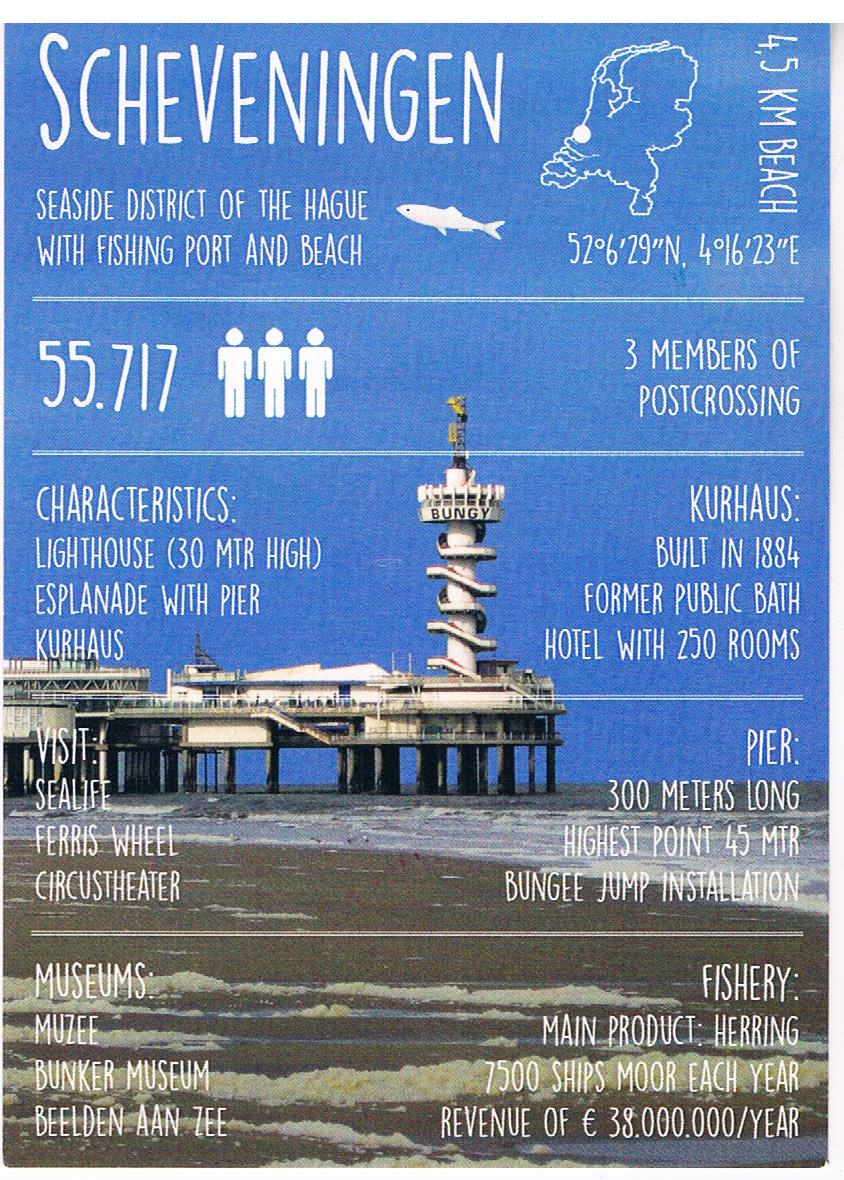The image features a detailed educational flyer against a backdrop of Scheveningen, the seaside district of The Hague. The foreground text overlays a scenic view of a unique pier architecture with a white tower labeled "bungee" and a tranquil beach with foamy ocean waves. The flyer provides comprehensive information about Scheveningen, noting its 4.5-kilometer beach, fishing port, and beach characteristics. Prominent landmarks highlighted include the 30-meter high lighthouse, the esplanade with the pier, Kurhaus built in 1884 with 250 rooms, and the 45-meter-high bungee jump installation. Other attractions listed are the Sea Life, Ferris Wheel, Circus Theatre, Museums, and the Musee Bunker Museum. The right side of the flyer contains geographical coordinates and additional details about the area, such as significant economic contributions from its fishery, primarily herring, with 7500 ships docking annually generating a revenue of 38 million euros.